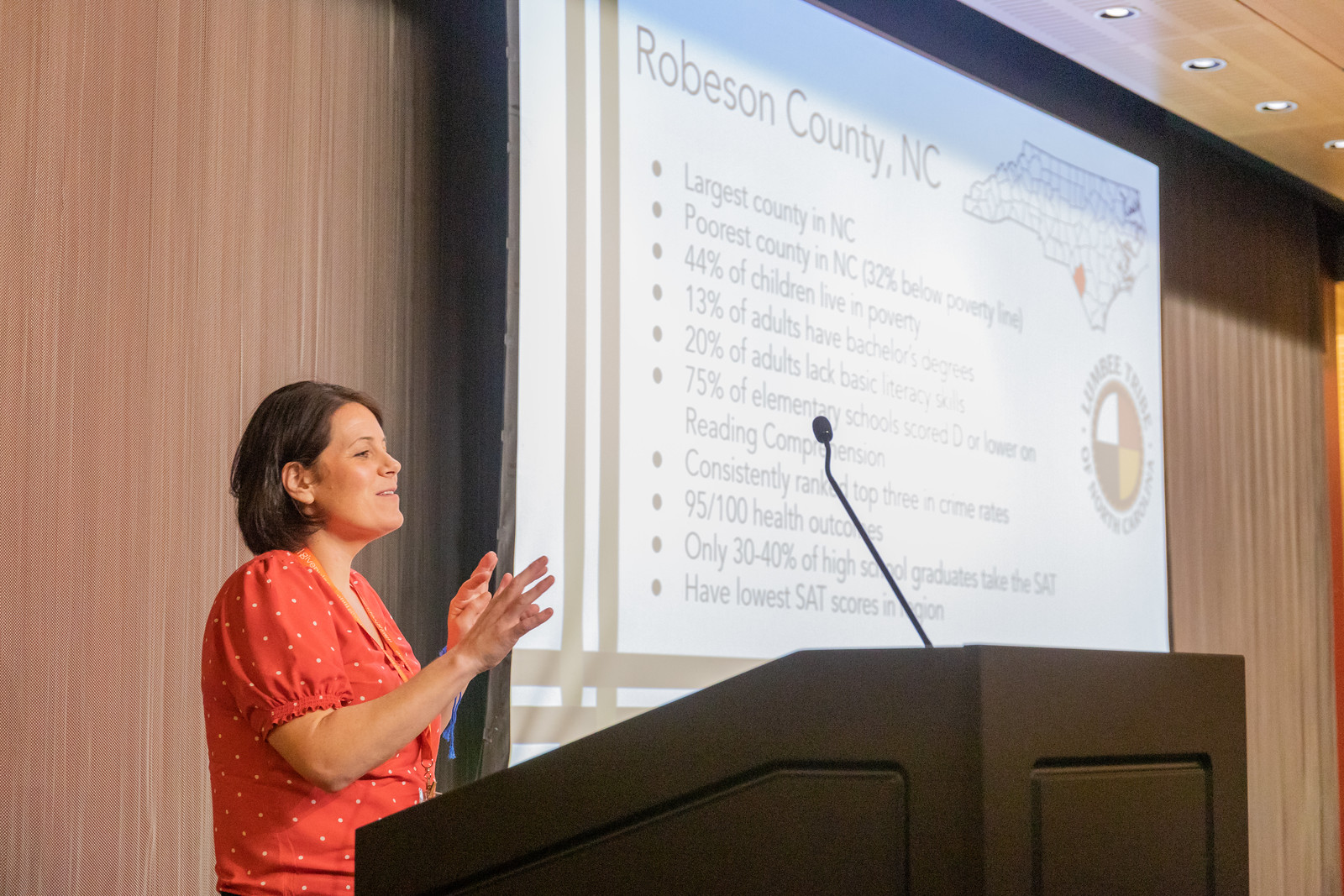In this image, we see a detailed indoor presentation setting, likely at a school. Dominating the lower portion of the image is a large brown podium with a microphone extending from its top. Standing to the left of the podium, a woman, who is evidently the speaker, addresses an audience. She has shoulder-length brunette hair and is dressed in a red top, complemented by a red or possibly orange lanyard around her neck. The woman is actively gesticulating with her hands as she speaks.

Behind her, a wood-paneled wall, which might also be a curtain, sets the background. To her right, a centrally positioned projector screen displays a presentation. At the top of the screen, bold text reads "Robeson County, North Carolina," accompanied by a small map highlighting the county. The presentation includes a comprehensive, bulleted list of socio-economic statistics about Robeson County, such as it being the largest and poorest county in North Carolina, with 44% of children living in poverty, and only 13% of adults holding bachelor’s degrees.

Additional points on the list detail that 20% of adults lack basic literacy skills, 75% of elementary schools score D or lower on reading comprehension, the county consistently ranks in the top three for crime rates, and it is 95th out of 100 in health outcomes. Furthermore, it states that only 30 to 40% of high school graduates take the SAT, yielding the lowest SAT scores in the region. The color palette of the image is diverse, featuring shades of light brown, brown, tan, pink, white, black, light blue, orange, yellow, and red.